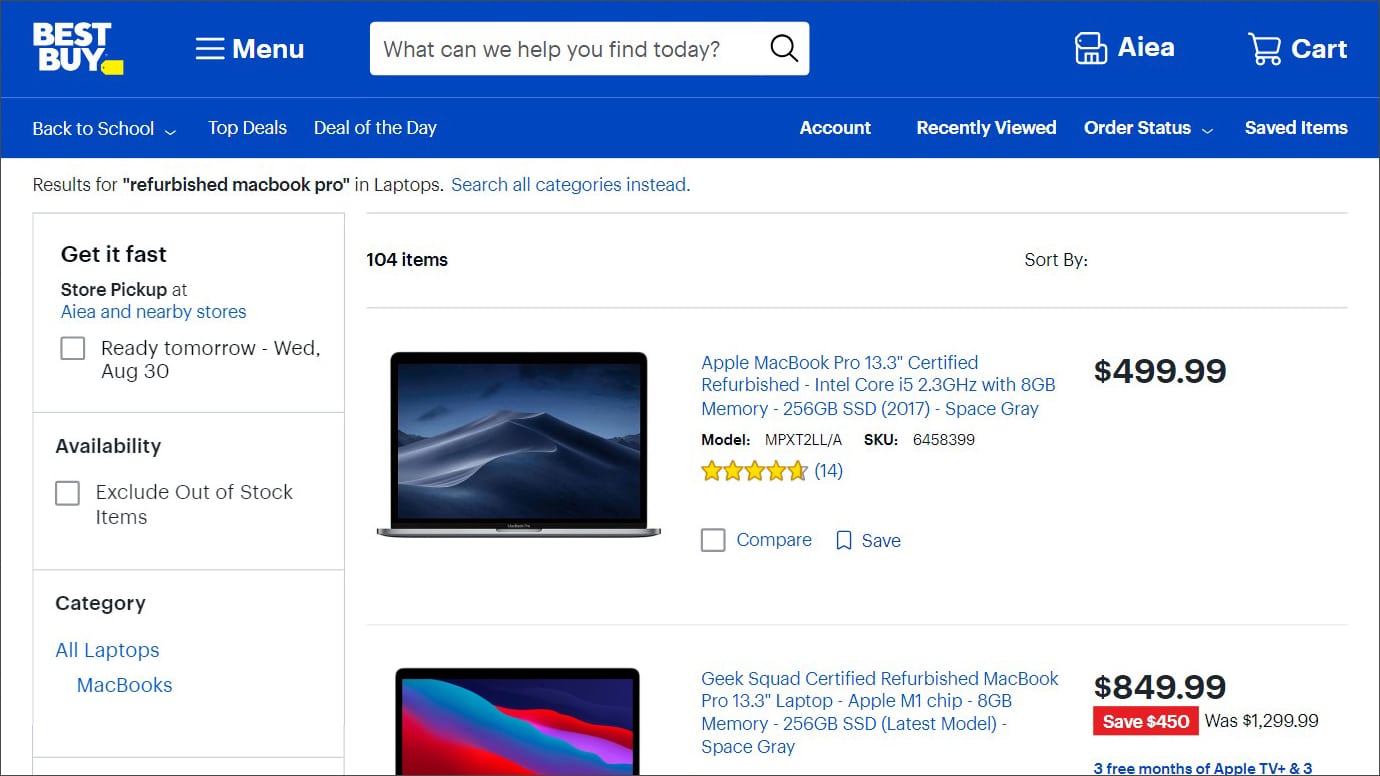The screenshot portrays the Best Buy website on a laptop or tablet. In the upper left-hand corner, the iconic "Best Buy" logo is showcased in bold white letters, accompanied by a yellow price tag attached to the "Y." Adjacent to the logo are three horizontal lines labeled "Menu." To the right is a search box with the prompt, "What can we help you find today?" and a magnifying glass icon. Further to the right are two icons labeled "AIEA" and "Cart."

Below these elements, a navigation bar displays several options: "Back to School" (with a dropdown menu), "Top Deals," "Deal of the Day," "Account," "Recently Viewed," "Order Status" (with a dropdown), and "Saved Items." Beneath this bar, the search result heading reads, "Results for 'refurbished MacBook Pro'," specifically in the laptops category, with an option to "search all categories instead."

The page shows that there are 104 items available. There are sections for "Get it Fast: Store Pickup at AIEA and nearby stores, ready tomorrow, Wednesday August 30," with a checkbox for selection. "Availability" offers another checkbox for "Exclude out of stock items." The "Category" filter lists "All Laptops" and "MacBooks."

On the right side, there are two visible product listings. The first item features a MacBook Pro with a 13.3-inch display showing an image of white sand dunes against a dark dusk sky. The description reads, "Apple MacBook Pro, 13.3 inch, certified refurbished," including details about the Intel Core and memory specifications. It has an almost five-star rating from 14 reviews and a price of $499.99. The product also features a "Compare" box and a "Save" ribbon for user selection.

The top half of the next featured laptop is partly visible, displaying a red and blue waves image that looks cloud-like. The description starts with "Geek Squad, certified refurbished MacBook," priced at $849.99 with a $450 discount from its original price of $1,299.99. The listing notes a three-month complimentary subscription to Apple TV.